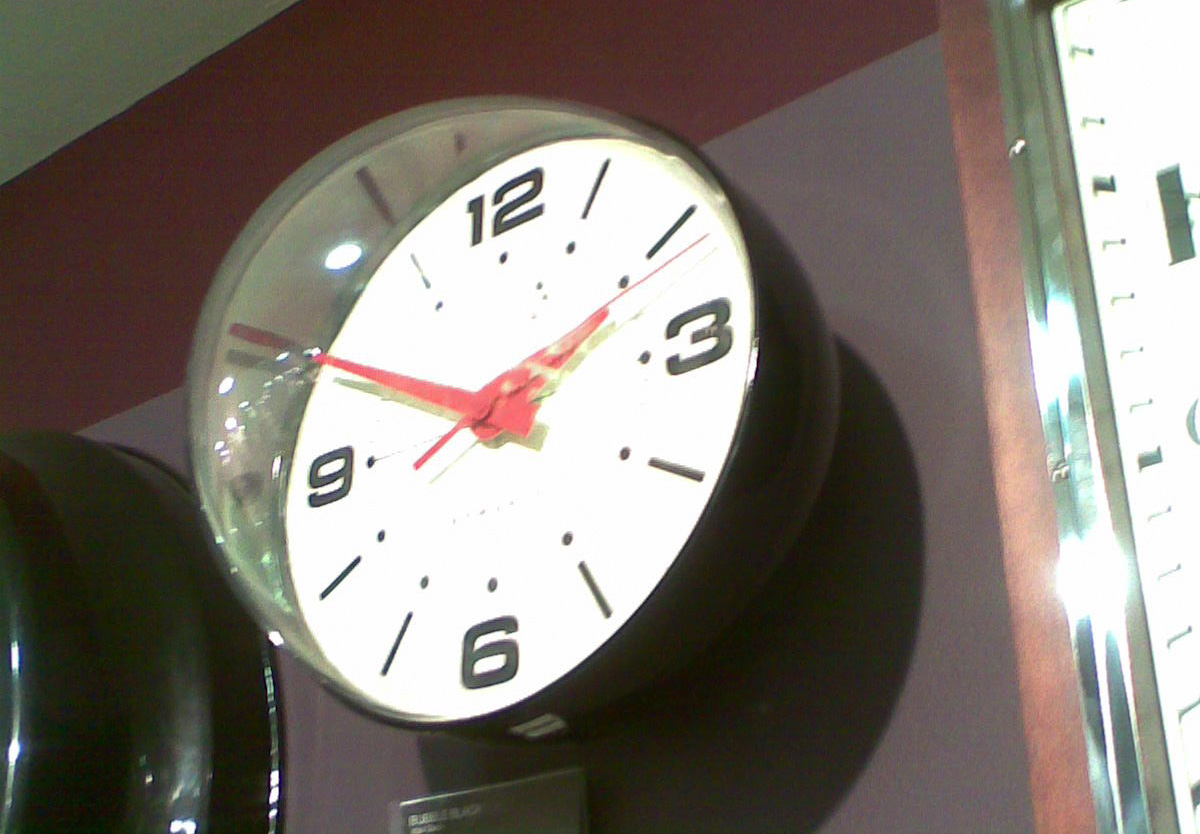The image depicts a wall-mounted, analog clock with a distinctive spherical glass cover, giving it a half-globe appearance that protrudes three-dimensionally. The clock face is white, featuring black numbers only at the 12, 3, 6, and 9 positions, while the intermediate hours are marked by black slashes and small black dots. The hour, minute, and second hands are red, with the hands showing a time of approximately 2:50, and the second hand pointing to roughly 13 seconds. Below the clock, there appears to be a sign, possibly indicating the name of a city. The clock is mounted on a wall and situated near another similar clock on the left, though this second clock is only partially visible. To the right of the clock, a shiny chrome strip, possibly part of a door or a blackboard frame, reflects light.